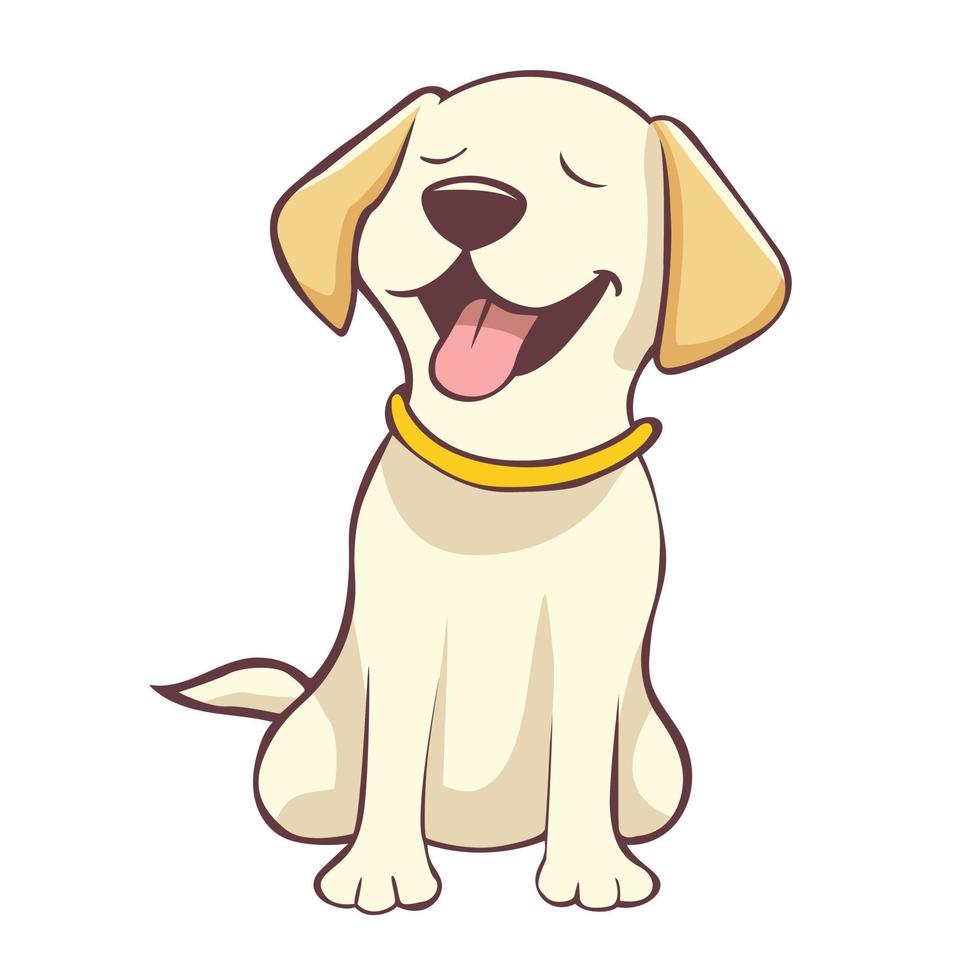This digital illustration depicts a cartoon dog sitting upright on its hind legs with its front legs extended. The dog, an ivory-colored puppy with fluffy, light brown ears laid flat, is portrayed with a cheerful expression. Its large brown nose and slightly smiling, open mouth reveal a friendly, pink tongue sticking out, giving the impression that the dog is yawning. The dog's eyes are closed, adding to its relaxed demeanor. It wears a yellow collar around its neck, and its short tail peeks out from behind its body. The image is detailed with a thick outline around the dog's features, and subtle shading adds depth to the character.